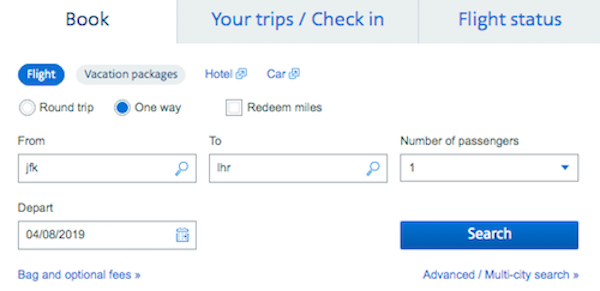The image depicts a user interface from a travel website, likely for booking a flight or vacation. At the top, there's a navigation bar with three tabs: "Book" (highlighted in white), "Your Trips/Check-In," and "Flight Status" (both in blue text and grayed out). Below, there are options for selecting "Flight" (highlighted in a blue button), "Vacation Packages" (grayed out), and "Hotel" and "Car" as additional selectable options.

Further down, the interface offers trip choices with radio buttons for "Round Trip," "One Way," and "Redeem Miles," where "One Way" is selected with a blue dot. Flight details include "From: JFK" and "To: LHR" with the number of passengers set to one, selectable via a drop-down menu while the departure and destination airports are entered through search bars. In the lower left corner, the departure date is set to "04-08-2019."

Additional options are noted, such as "Bag and Optional Fees." At the bottom is a blue search button with "Search" in white text, next to a link for "Advanced/Multi-City Search."